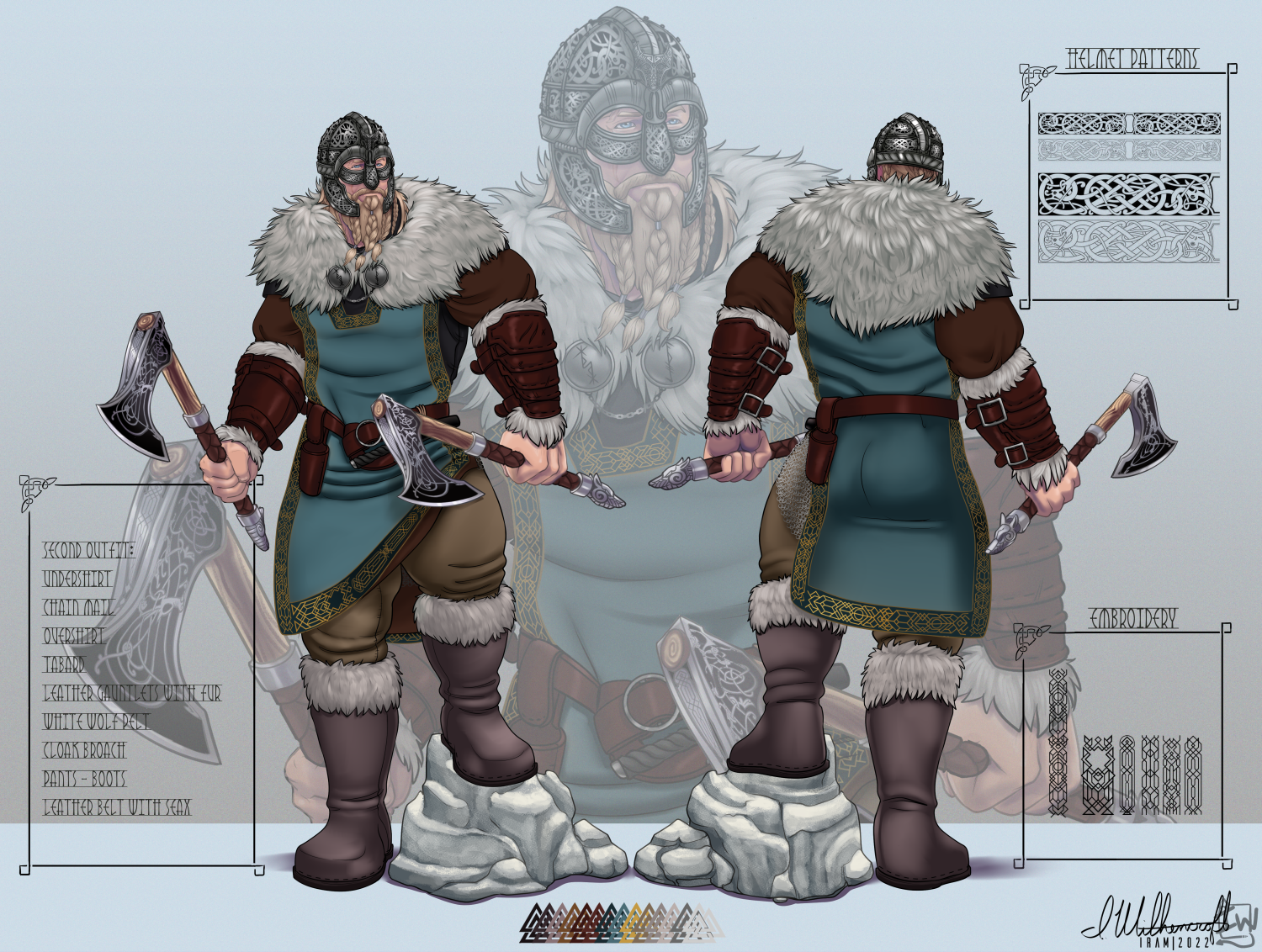This image is a detailed piece of concept art depicting a Viking warrior, illustrating the character from various angles and emphasizing specific design elements. The central focus includes two prominent poses: a frontal and rear view of the Viking, with a larger, semi-transparent rendition of him in the background.

The Viking is dressed for winter, wearing a metal helmet that shields his head, eyes, and cheeks. His fair skin is complemented by a blonde braided beard, and he sports a large, fluffy white fur collar. The tunic he wears is blue with gold embroidery and hangs over a brown undershirt. His sleeves are protected by brown armor, and he clutches a pair of large, silver-headed axes with brown wooden handles.

His lower attire includes big, heavy brown fur boots, and he is depicted placing one foot on a stone. Surrounding the character are various annotations and artistic notations. In the top right corner, there are repeated helmet patterns labeled "helmet patterns." The bottom right corner features black and white line drawings labeled "embroidery," and a slightly indecipherable artist's signature dated 2022.

Additionally, the bottom left corner contains a descriptive box detailing a second outfit, which includes an undershirt, chainmail, overshirt, tabard, leather gauntlets with fur, white wolf pelt cloak, brooch, pants, boots, leather belt with SAX (seax), and corresponding color patterns.

The background of the entire image is blue, enhancing the contrast and clarity of the Viking character and the intricate details of his attire and weaponry. The artwork combines a demonstration of helmet designs and embroidery patterns, emphasizing the historical and artistic elements of the warrior's appearance.